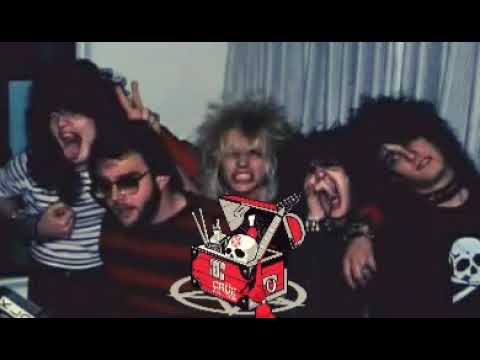This photograph captures an 80s rock band, likely Motley Crue, known for their big hair and heavy metal style. The five band members are aligned closely, leaning on each other. Notably, they display an array of expressive poses: some are yelling with mouths wide open, others grimacing, and one member remains expressionless. Their distinctive hairstyles range from spiky to long and voluminous, embodying the iconic 80s look.

The man on the far right stands out with a skull depicted on his black shirt, while another on the left has a tongue sticking out mischievously. One band member with a striped red and black shirt and sunglasses sports a shorter hairstyle and a beard. The background features a white wall, a door with light filtering through, and a silver curtain covering a window.

In the foreground, a detailed cartoon graphic showcases a vibrant red treasure chest outlined in white. Inside, there are skulls, a guitar, drumsticks, and a bottle of Jack Daniels, all symbolizing rock ethos. The chest is perched atop a pentagram, lending the image an edgy, potentially satanic rock band ambiance.